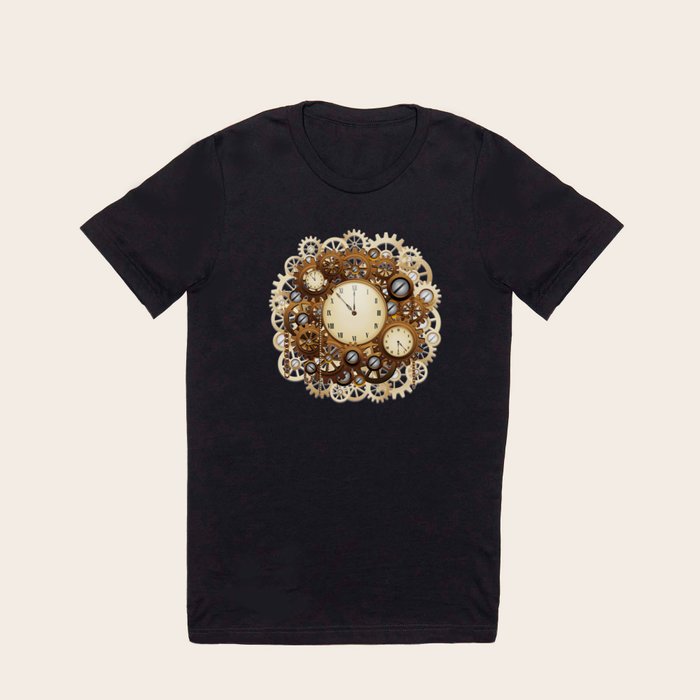This image showcases a stylish black shirt adorned with a striking design at its center. Dominating the design is a white clock face bordered by a detailed copper rim, displaying the time at approximately 11:49 or 11:50. Behind the clock, intricately arranged gears add depth and complexity to the artwork, possibly symbolizing the relentless passage of time. The shirt, lying flat against a clean white background, emphasizes the vividness and intricacy of the clock and gears, making them the focal point of this engaging visual piece.